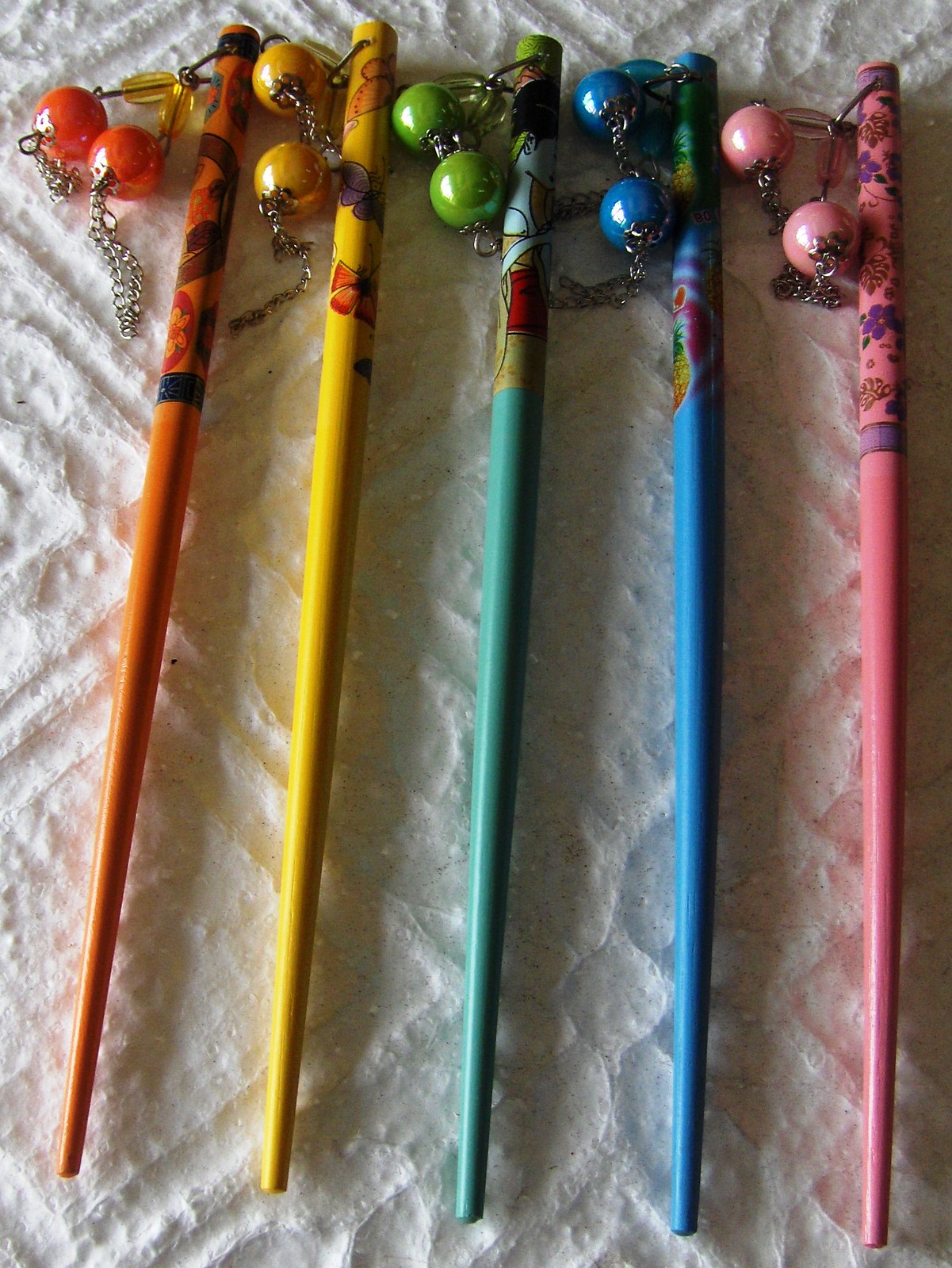The image in portrait mode captures a close-up of five pencil-like but not pencil objects that are resting vertically on a textured white surface, possibly anaglypta wallpaper or a tablecloth. These slim, wooden poles—resembling chopsticks or slender musical instruments—are decorated with intricate patterns near their tops. From left to right, their colors are orange, yellow, green, blue, and pink. Each has floral or butterfly designs, with the orange one possibly featuring a woman’s depiction. At the end of each pole, a string attaches two baubles with silver chains hanging from them, matching the color of the respective pole: orange, yellow, green, blue, and pink. Their width is about half an inch and they appear to be designed to produce sound when shaken, with the baubles creating noise upon contact with the poles.